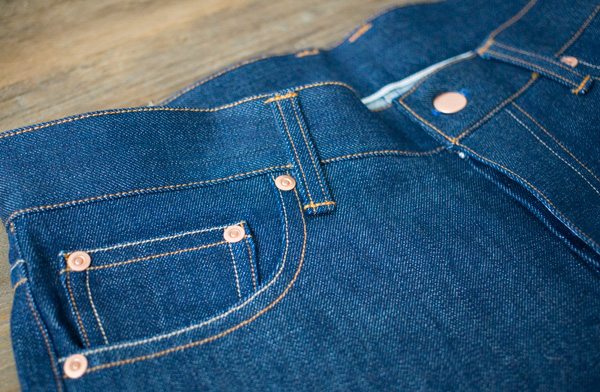The image showcases a vibrant blue pair of brand new jeans laid on a light brown wooden surface, which appears to be a table or possibly a wood-planked floor. The wood has a natural finish with signs of wear and tear, adding a rustic charm. The jeans are made of soft, stretchy cotton denim and feature contrasting gold stitching along the waistband, pockets, and belt loops. The design includes a prominent copper-colored button at the waist, accompanied by a zipper. Only a portion of the jeans is visible, highlighting the right main pocket and the smaller watch pocket inside, although no tags are within view.